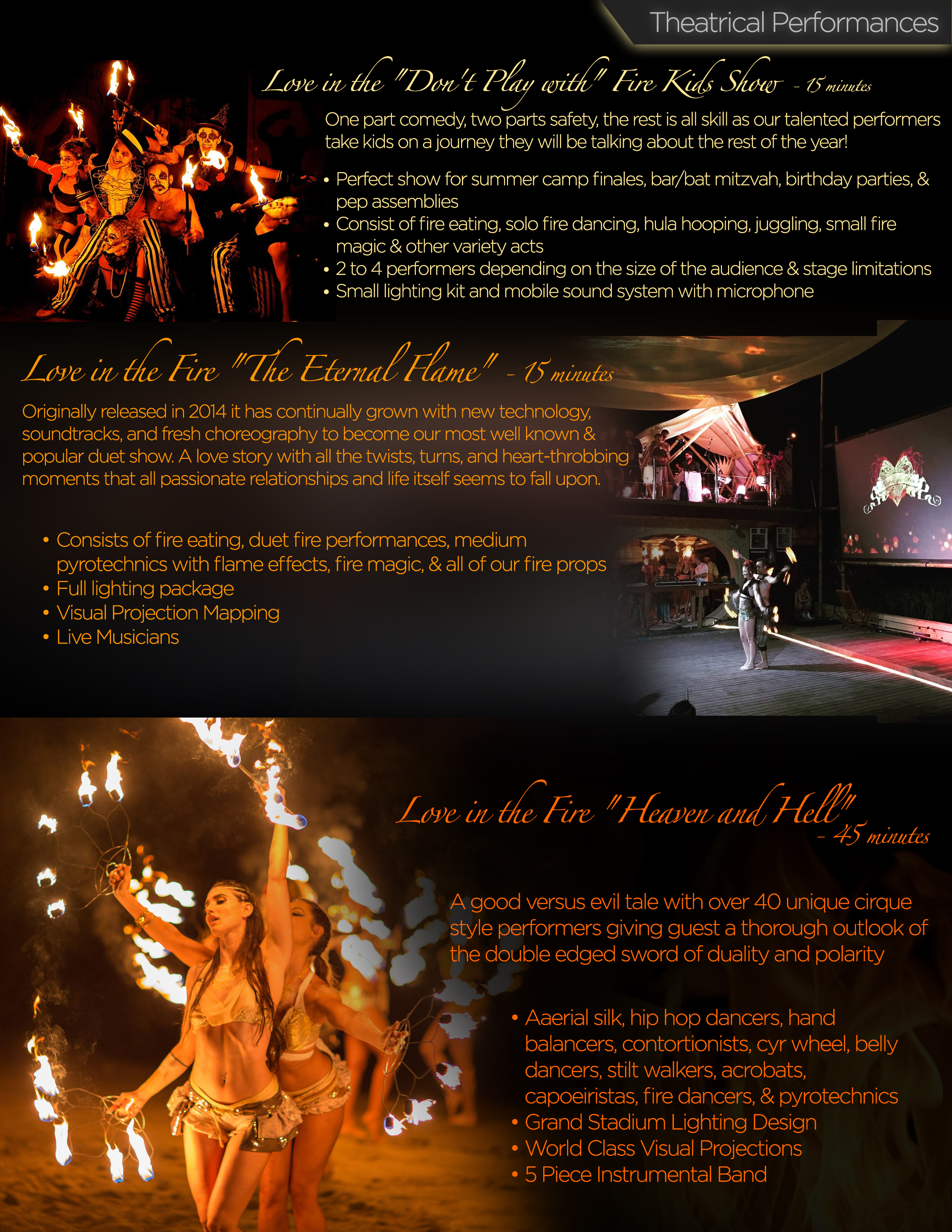This image, set against a black background, serves as an advertisement flyer for a series of theatrical performances. At the top, it is labeled "Theatrical Performances" in white text. The flyer features three performances, each accompanied by a photograph and a brief description.

The first performance, titled "Love in the Don't Play with Fire Kids Show," lasts 15 minutes. The photograph shows a group of people in clown makeup holding torches. The description highlights that the show is "one part comedy, two parts safety," focusing on educating children about safety in an engaging and memorable way.

The second performance is "Love in the Fire: The Eternal Flame," also 15 minutes long. The accompanying image is of a dynamic stage scene, illustrating the intense and mesmerizing fire-eating duet that defines this show.

The third performance, "Love in the Fire: Heaven and Hell," runs for 45 minutes. This segment is depicted with a photo showing a dramatic good versus evil tableau, aiming to portray a riveting narrative of moral and elemental conflict.

Each performance is visually represented to provide a glimpse of the energy and themes explored, making this flyer a striking and informative piece to attract potential audience members.